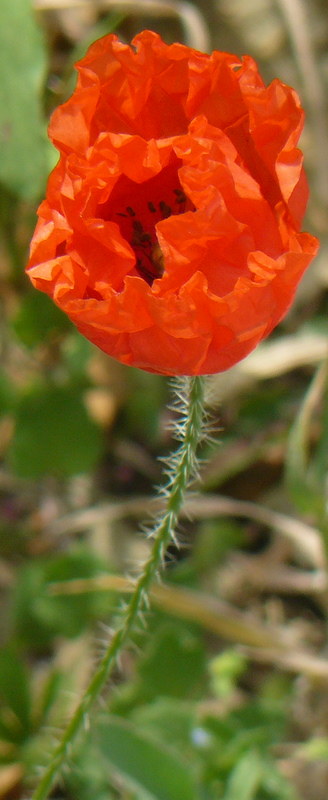This close-up, color photograph, in a narrow vertical portrait orientation, showcases a blooming red California poppy. The vibrant orange-red petals, arranged in ruffled concentric circles, are beginning to open, revealing a partially visible center sprinkled with black seeds. The flower is held by a thin, angled stem, adorned with small, prickly barbs and white hair-like structures. The background features a soft blur of green and beige foliage, creating a natural, yet undefined setting that could range from a backyard to a wild field or forest edge. The artistic style of the photograph is photographic representationalism realism, capturing the detailed textures and colors of the flower while leaving the context open to viewer interpretation. The image has no people, text, title, or specified location, highlighting the delicate intricacy of the poppy against its softly blurred backdrop.